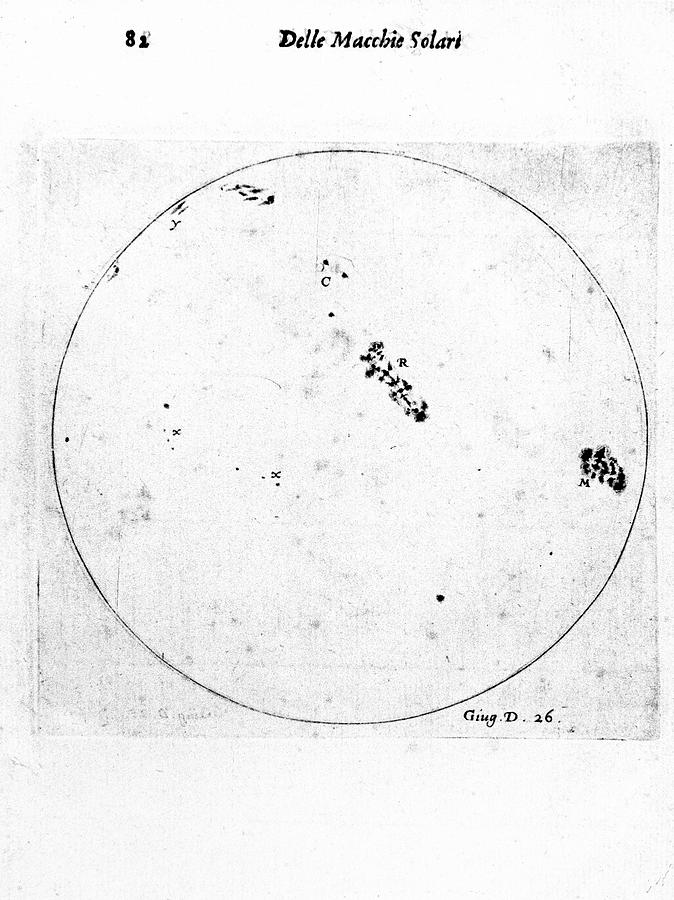The image depicts an old, textured gray and white background featuring a prominent sphere or planetary-like circle with distinct black markings inside. Above the sphere, the top left corner displays the number '81'. Centered above the sphere are the words "Del Macchie Solari," spelled variously but commonly as D-E-L-L-E space M-A-C-C-H-I-E space S-O-L-A-R-I. Within the sphere, various black line markings are scattered, resembling an intricate pattern viewed under a microscope, including a notable cluster towards the right side and several patches around its surface. Below the sphere, towards the bottom, the text "G-I-N-G dot D dot 26" (alternatively seen as G-I-U-G dot D dot 26) is inscribed, adding to the antiquated and scholarly appearance of the image.